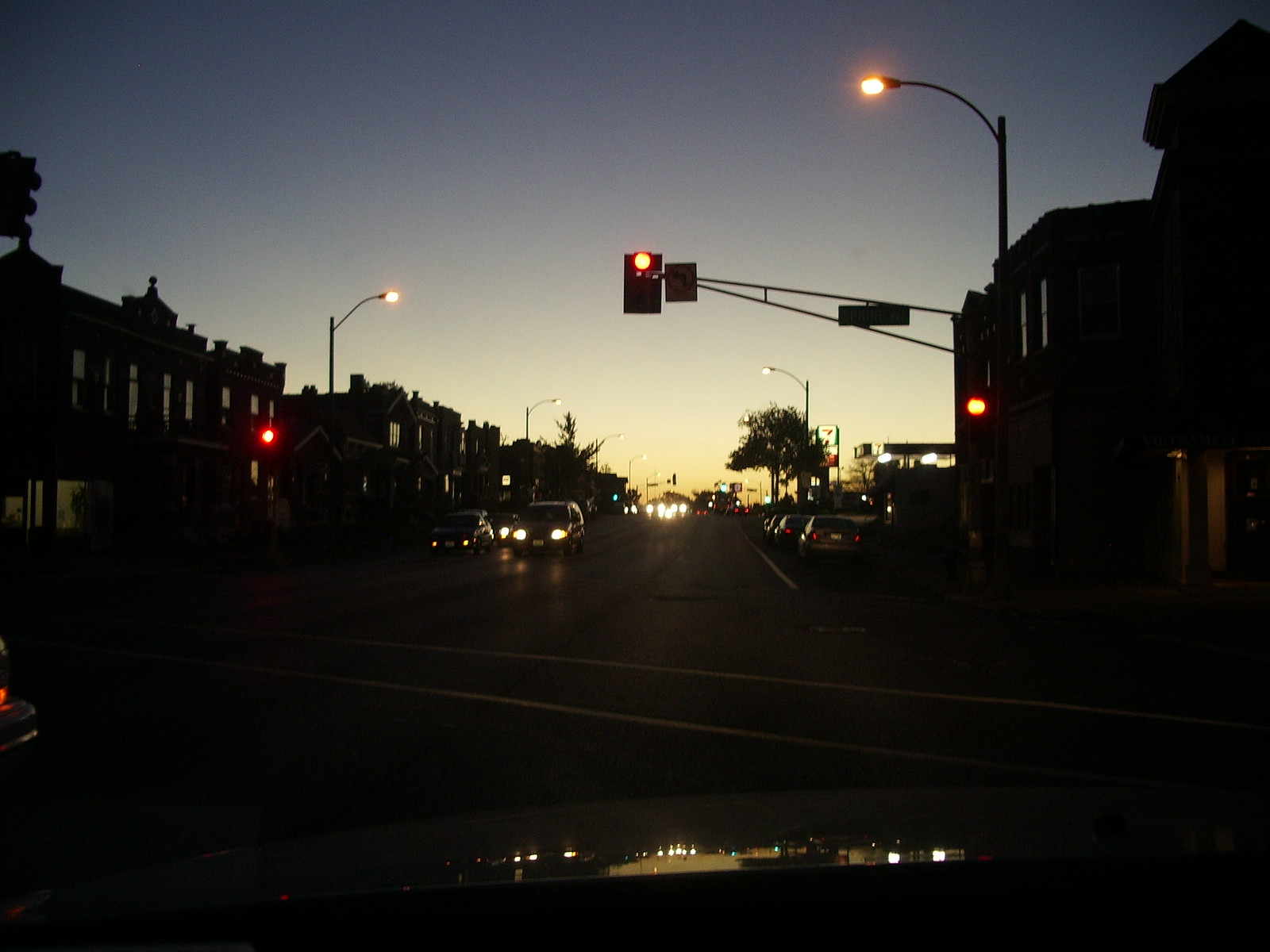This photo, captured from the driver's perspective through the front windshield of a car stopped at a traffic light, offers a detailed glimpse down a bustling street at dusk. On the left side of the street, two-story, antiquated buildings line the road, their aged facades subtly illuminated by the fading daylight. The oncoming traffic on this side adds a dynamic element to the scene. To the right, several cars are parked, their taillights brightly reflecting off the car's headlights. Further down on the right, an awning of a gas station is visible in the distance, adding a touch of modernity. The sky above is transitioning from blue to dark, indicating the approaching night, while the horizon in the center of the photo is tinged with an orange hue from the setting sun.